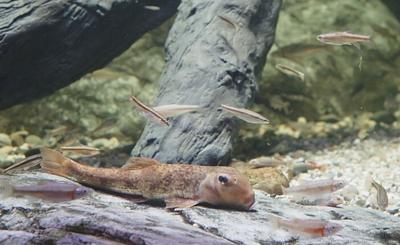This intricate underwater photo captures a serene, yet complex scene. Dominating the lower part of the image is a brown suckerfish with a slightly yellow tinge and a speckled pattern across its back. The fish, which almost seems as if it could be a land creature, is lying atop what appears to be a gray, ridge-edged log. This log intersects with another vertical log behind it, adding a layered depth to the scene. The facial features of the suckerfish are distinct, with a black eye and a mouth located underneath its face, giving it a unique appearance. Surrounding the main fish are six small, minnow-like fish that swim against a blurred, predominantly green but partly gray forest-like background, lending the scene an almost mystical, composite quality. To the right of the fish, there's a gray rock with textured ridges. The overall setting, possibly an aquarium, adds to the visual interest with elements like scattered gravel and multiple fish swimming around, contributing to a captivating underwater vignette.